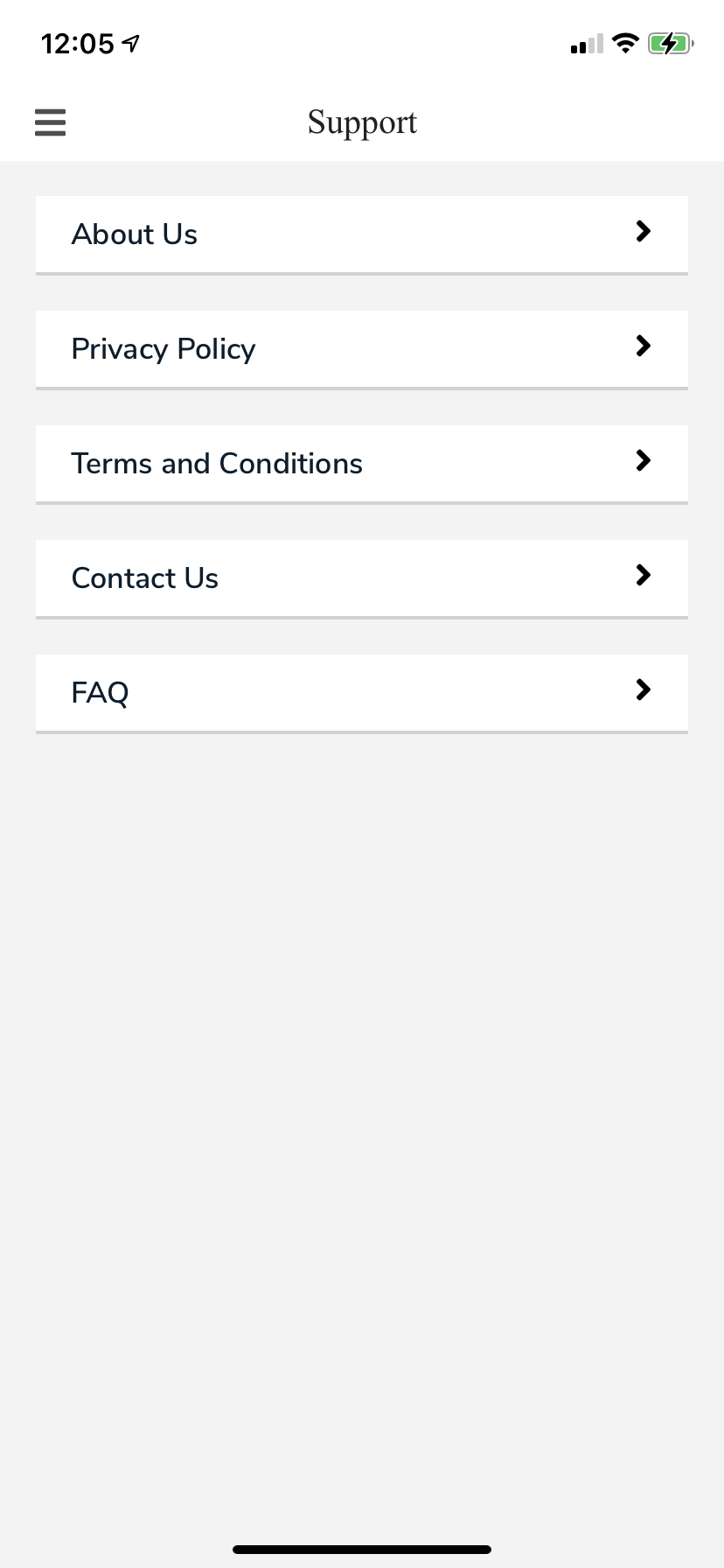Screenshot of a mobile phone displaying the "Support" section. At the top left corner, the time is shown as 12:05. In the top right corner, there are icons for cell phone signal, Wi-Fi signal, and battery status, with the battery icon in green and a lightning bolt graphic indicating charging. The page title, "Support," is prominently displayed. Below the title, there are five distinct rows, each contained within its own white bar and separated by uniform gray spaces. The text within each bar is black. The rows are labeled as follows: "About Us," "Privacy Policy," "Terms and Conditions," "Contact Us," and "FAQs." Each row also features a right-pointing arrow at the end. The overall background of the screenshot is gray.